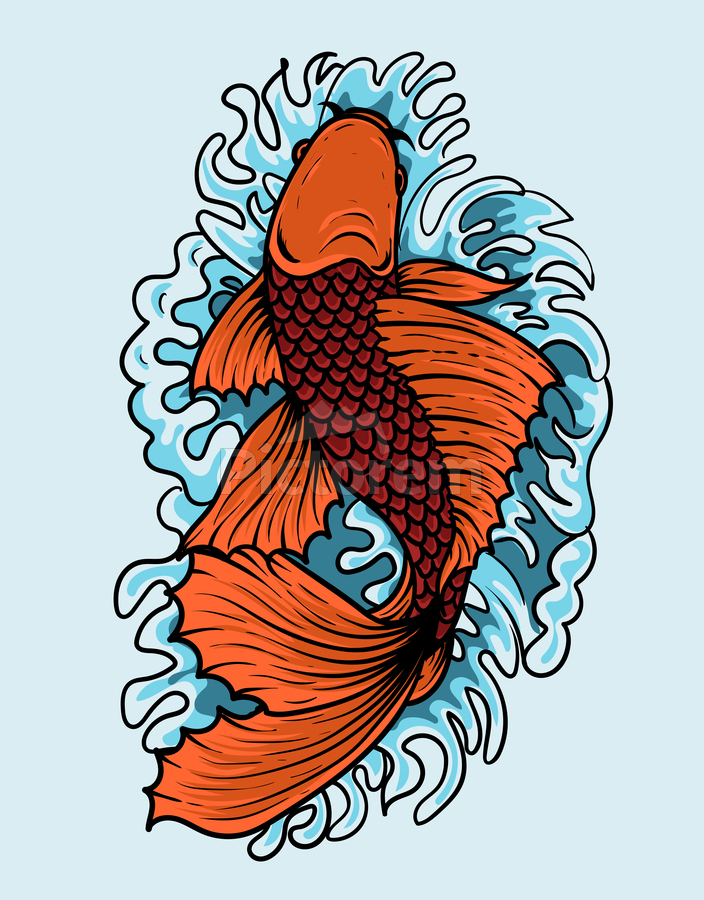The illustration depicts a striking koi fish, viewed from directly above, gracefully curving its body in an S-shape as it appears to splash through water. The fish's body is covered in tiny, burgundy-red scales highlighted with black outlines, while its long, broad fins and its head are a vibrant orange. Poking out from the fish's mouth are small, pointed feelers, and its large, protruding eyes add to its expressive appearance. Surrounding the fish are dynamic patterns of dark blue and light blue waves, outlined in black, creating an impression of motion and splashes. The entire scene is set against a light blue background, which subtly features the faint text "Picto-M" overlaid on the image.